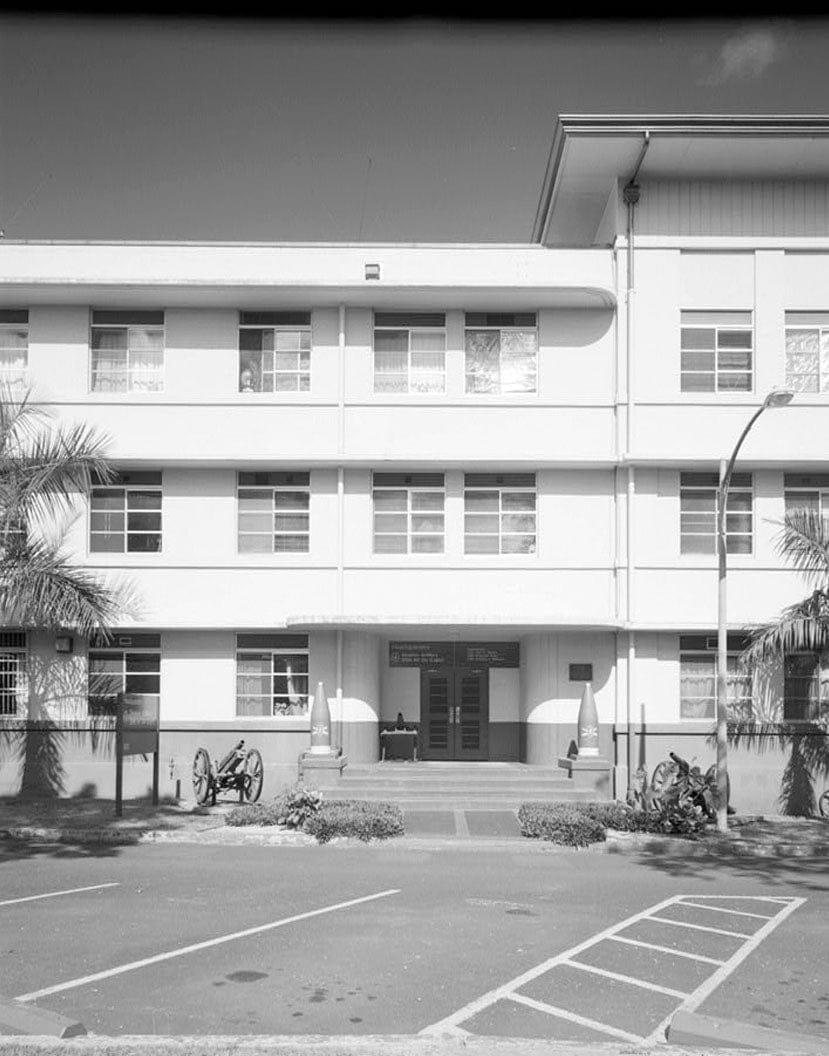The image displays a three-story, Art Deco-style building, potentially a historical or government site. The black-and-white photograph suggests the building is relatively white, characterized by its horizontal design and wide window insets arranged in a two-by-three grid with an additional cap window extending towards the ceiling. The entrance, reached by a short staircase of about four steps, is flanked by two old-looking cannons with large wheels. Above the entrance, which features two wooden French doors, there is a sign with some writing, though the details are unclear. On either side of the building, there are palm trees, hinting that the location could be in Florida or the Caribbean. The building is set against the backdrop of a parking lot, adding to the scene's tranquil ambiance.